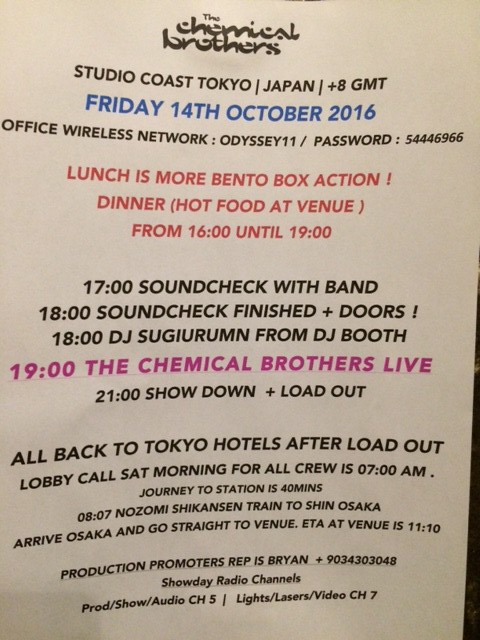The image showcases a detailed printed schedule for a Chemical Brothers concert at Studio Coast in Tokyo, Japan, dated Friday, October 14, 2016. The document, intended for crew members, includes critical logistical details in a clear and organized format. Key events, such as the live performance by the Chemical Brothers, are highlighted in red text, while other information is presented in black. The schedule starts with soundchecks at 17:00, with DJ Sugurun performing from the DJ Booth at 18:00. The Chemical Brothers take the stage at 21:00, followed by loadout and instructions for the crew to return to Tokyo hotels. Meals provided include bento boxes for lunch and hot food at the venue from 16:00 to 19:00. The schedule also lists office wireless network details, a contact for production promoter reps, and show day radio channels. The layout employs different colors to emphasize important sections, enhancing clarity for crew navigation.